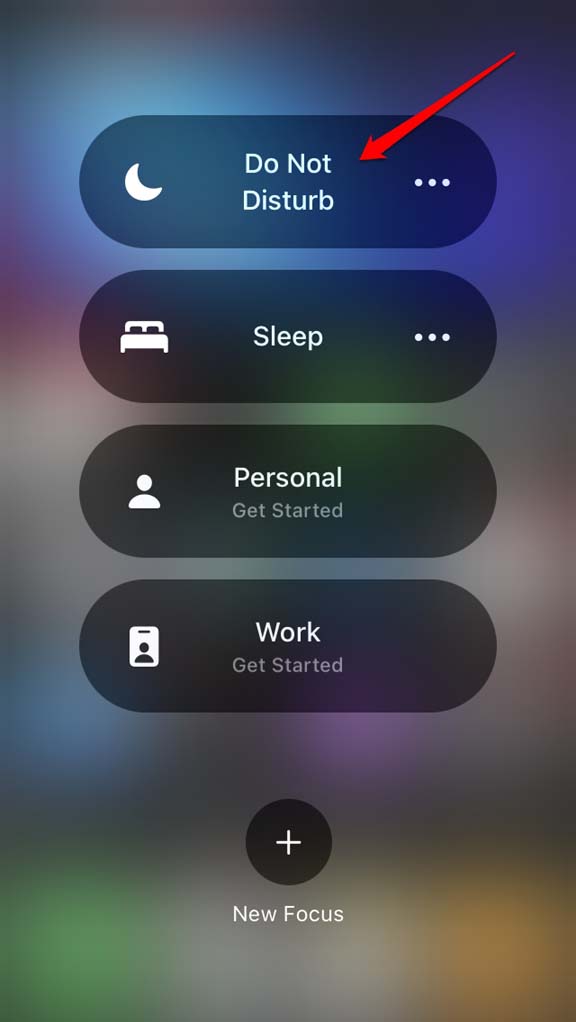The image showcases multiple screenshots of an iPhone's Control Center, specifically highlighting the Focus tab. A prominent red arrow points towards the "Do Not Disturb" option, drawing attention to its importance. Also visible in the Focus tab are other options including "Sleep," "Personal," and "Work," each accompanied by a "Get Started" prompt. Additionally, there are buttons labeled "New Focus" and "Add New Focus" for creating custom settings. The background of the image is heavily blurred, with a mix of colors such as blue, green, purple, red, and gray, adding a vibrant yet subtle ambiance to the scene.